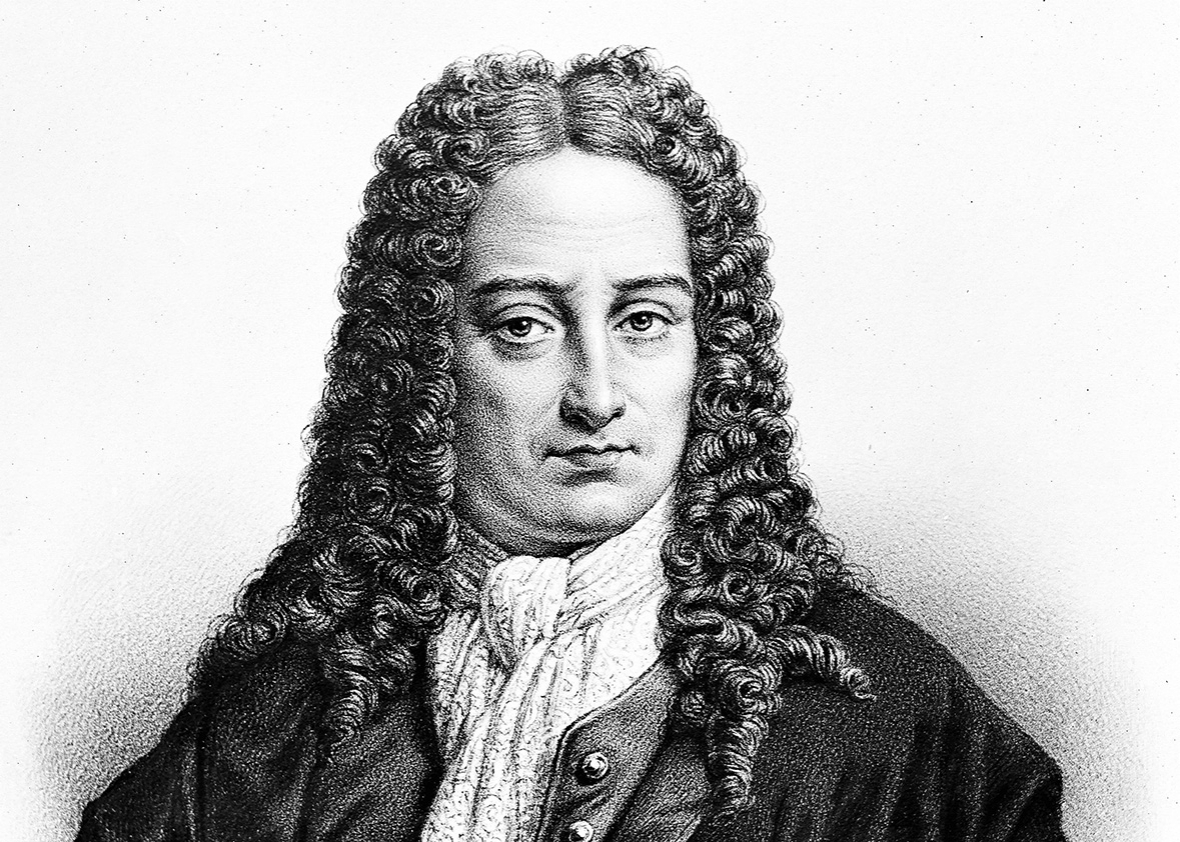This detailed etching presents a monochromatic portrait of Gottfried Wilhelm Leibniz, a renowned mathematician and contemporary of Isaac Newton. The gentleman depicted is adorned in long, flowing ringlets of dark hair, likely a wig common in that era. He is dressed in a traditional coat over a white shirt, which features a wrap-around neck covering rather than a modern necktie. The coat is unbuttoned, revealing a sense of relaxed formality. His gaze is direct and neutral, neither smiling nor frowning. The hair cascades over his shoulders, adding an air of sophistication to the composition. This etching captures Leibniz's thoughtful demeanor, underscoring his intellectual legacy in the realm of calculus and philosophy.